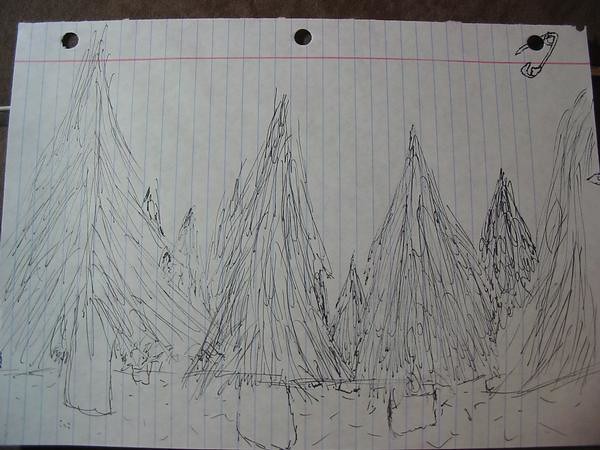The image is a photograph of a piece of lined notebook paper oriented sideways with the three punched holes at the top. The paper features a detailed forest scene, possibly drawn with either pencil or pen. Across the length of the paper, several pine trees are sketched, resembling a dense pine tree forest. Some of the trees are very tall, reaching up towards the holes, while others are shorter and appear in the background. There is a mix of faint and dense shading, with some trees more prominently detailed than others. Specifically, one tall tree stretches almost to the top of the page, and beside this, various trees are partially visible, creating a layered effect. A unique feature is the small safety pin drawing integrated into the top right hole, giving the illusion of it being threaded through the hole. Additionally, the lined paper shows a red margin line running horizontally below the holes, with blue lines running vertically. In the background of the image, part of a person's face, including half an eye, ear, and hair, is faintly visible, adding an intriguing, almost hidden, human element to the scene. The paper itself rests on what appears to be a black table, just visible around the edges.